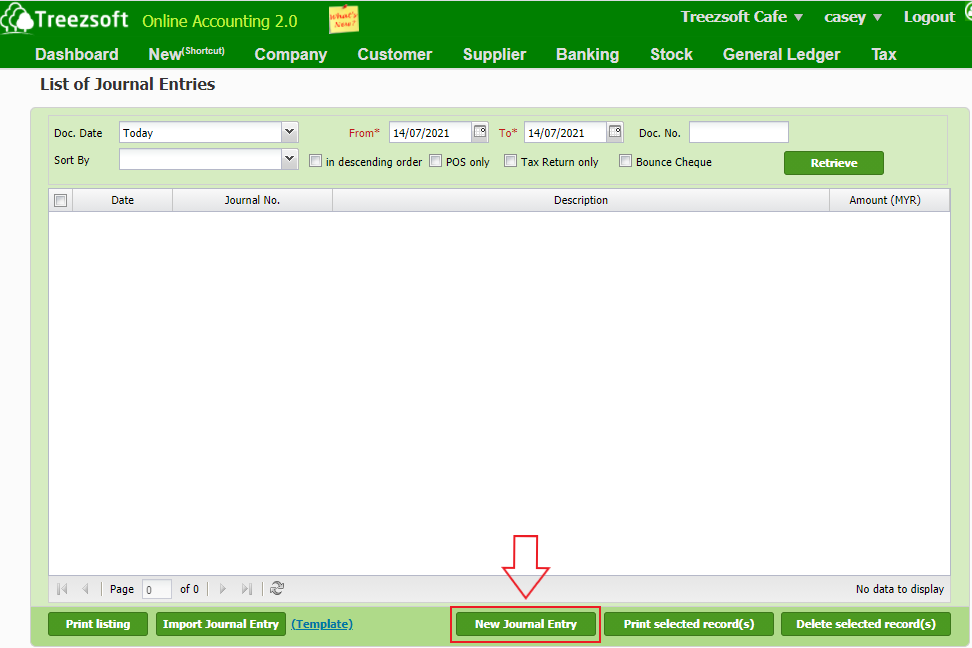Screenshot of a Treesoft App Interface:

The image captures a screenshot of the Treesoft app interface. The top border is green, serving as a menu bar featuring mostly white font. On the left side, the company's name, "Treesoft" (spelled T-R-E-E-Z-S-O-F-T) is displayed in white font with an icon of two trees adjacent to it. Next to it, in a yellow font, it reads "Online Account 2.0." On the right side of this green border, several buttons are displayed, including "Treesoft Cafe," the user name "Casey," and a "Logout" option.

Beneath the green border, there are several menu buttons, each labeled in white font: "Dashboard," "New Shortcut," "Company," "Customer," "Supplier," "Bank & Stock," and "General Ledger & Tax."

The central section of the screenshot is primarily white and lists journal entries, resembling an accounting journal. A white box contains the label "Document Date" (abbreviated as "D-O-C Date") in black font, currently set to "Today." Another white box labeled "Sort By" sits beside it, with a date range displayed as "14-07-21 to 14-07-20-21."

The interface also includes sections to input document numbers and sorting information. The lower section features a large green box containing smaller white boxes. 

At the very bottom of the app, there are several buttons: "Print List," "Import Journal Entry," and "New Journal Entry." An arrow points to the "New Journal Entry" button, indicating that this is the focal point of the screenshot.